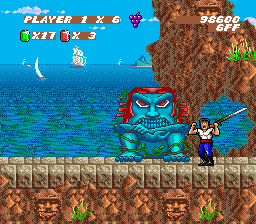This screenshot captures a heated moment from a video game in a classic 4:3 aspect ratio. Dominating the scene are two characters: the player and a formidable boss. The player character, a humanoid warrior, stands out in a white shirt, blue pants, and a red belt, wielding a gleaming sword. They are locked in battle against a giant stone monster, distinguished by its blue skin, menacing red eyes, and fiery red hair. The backdrop features a serene ocean with a solitary sailing ship on the horizon, adding depth to the intense scene. The ground they battle on is a rugged stone platform, beneath which lie dark golden, Egyptian-style heads embedded in what appears to be bedrock. At the top of the screen, player information is displayed, indicating "Player 1 x 6" lives remaining. Additionally, the score reads "98,600 6FF," adding a competitive layer to the thrilling encounter.